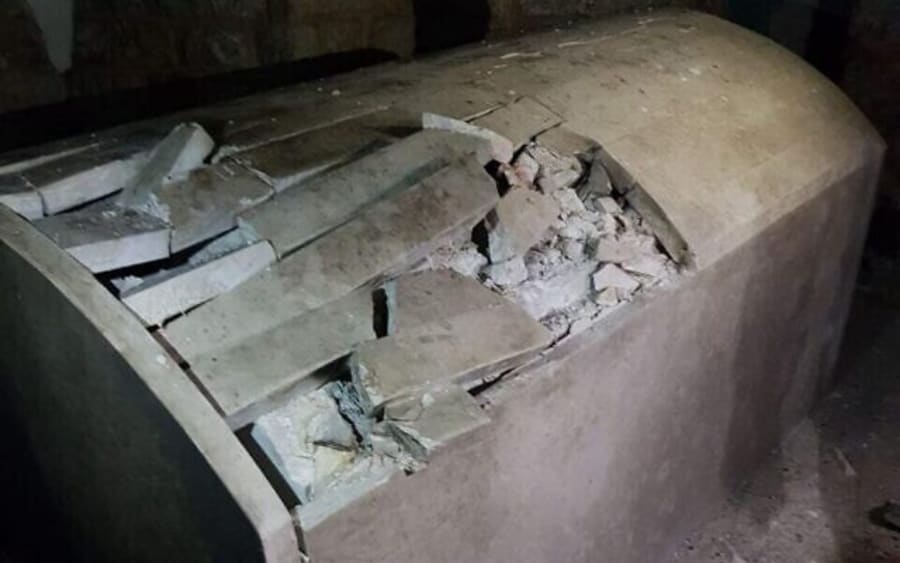The image depicts a close-up of a severely damaged concrete casket or tomb, resembling a stone mausoleum. The top of the structure has been violently broken open, revealing a jumble of crushed cement and broken concrete blocks. The casket is situated in a semi-dark, grainy environment, likely an underground or cave-like area, lending an eerie atmosphere to the setting. The surrounding room is characterized by its grayish-brown walls and floor, with a single light source illuminating the desecrated tomb. The remnants of concrete strips or segments are scattered across the top, indicating a deliberate attempt to break into the casket. Amidst the shadows, the faint outline of a man's hand suggests the presence of the photographer, casting an eerie shadow on the undisturbed portion of the tomb. The cause of the damage is unclear—whether it was due to vandalism, a natural disaster, or an archaeological excavation.